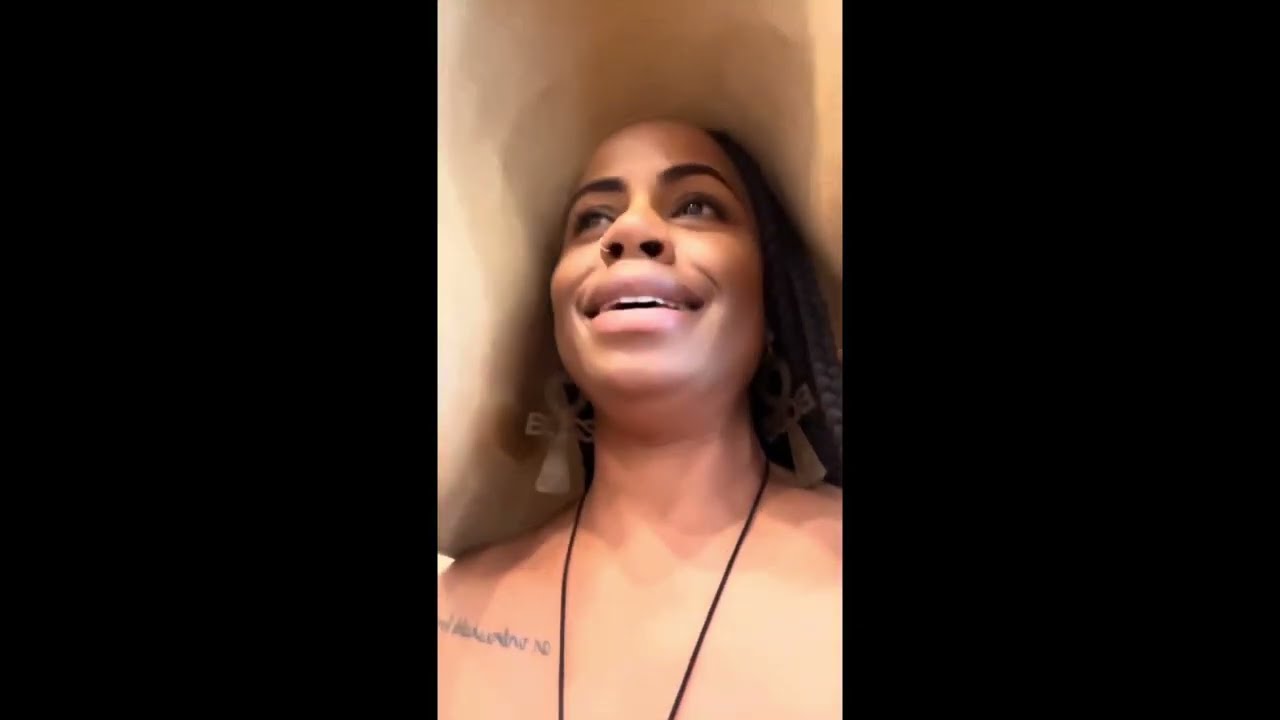The color photograph portrays an African-American woman captured from a low angle with her nostrils prominently visible. She gazes upward, her expression suggesting mid-speech or an emerging smile, with her lips slightly parted. Her striking features include thick, brown braids that cascade around her face, and she wears an elaborate brown sun hat casting shadows over her forehead, neck, and shoulders. Accentuating her appearance are large earrings shaped like onk crosses inscribed with the word "BOSS," and a black cord necklace adorning her bare chest. A tattoo featuring possibly Arabic writing decorates her right shoulder, adding to her distinct look. Her right nostril is pierced with a nose ring, and she is illuminated by a halo of light, with the overall scene framed by a thick black border.